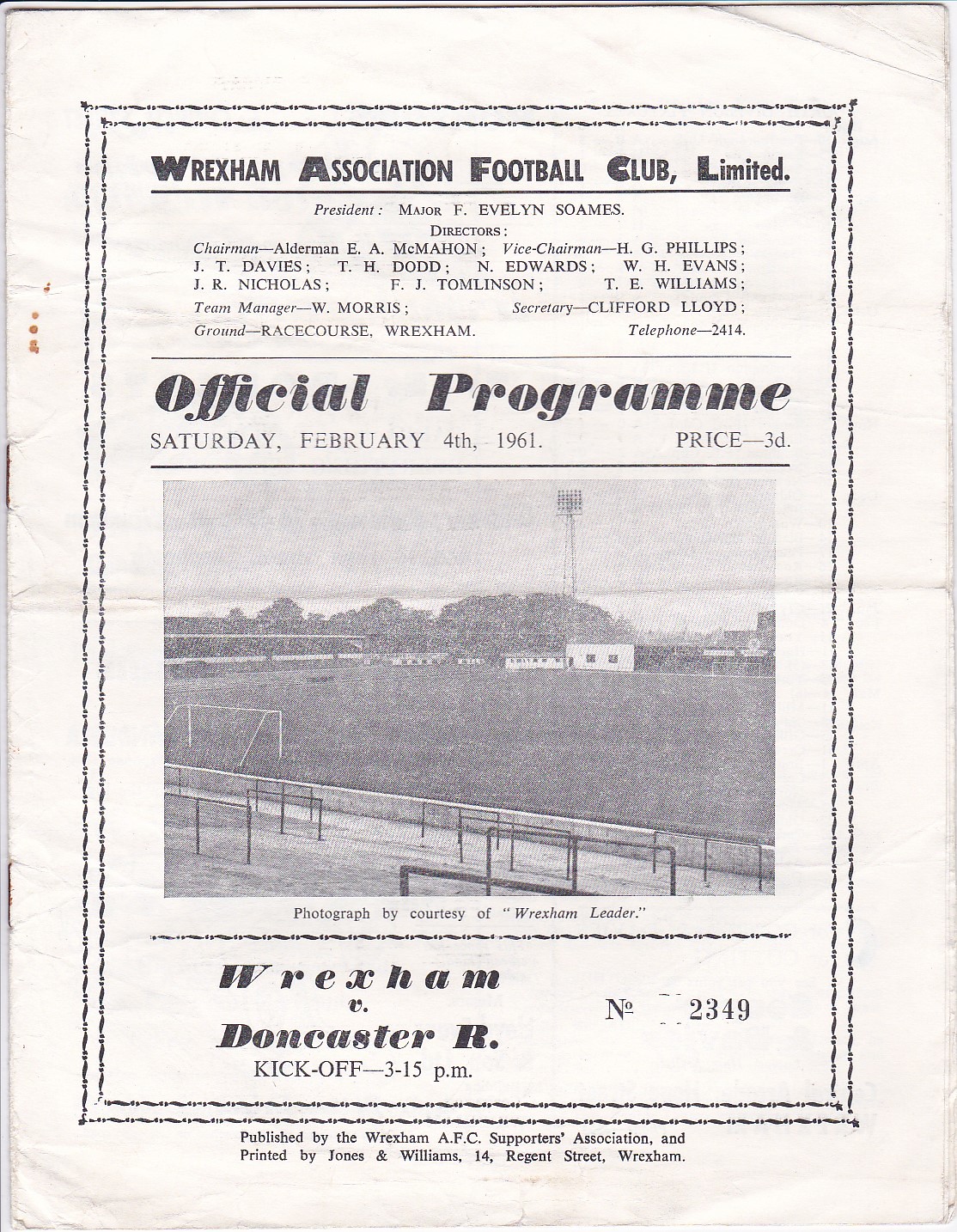The image is a vintage, black and white printed cover of an official program from the Rexham Association Football Club Limited, dated Saturday, February 4th, 1961, priced at 3D. The cover, which is faded and tattered with wrinkles and two staples on the left-hand side, features bold text at the top reading, "Rexham Association Football Club Limited," followed by a rule line and then "President: Major F. Evelyn Soames." Below this, there is a list of the directors in very tiny print along with chairman and vice-chairman names, including Aldermen McMahon, Phillips, Evans, Edwards, Williams, Dodd, Davies, Nichols, and Tomlinson. The team manager is W. Morris, and the secretary is Clifford Lloyd. The ground is listed as Race Course, Rexham, with a phone number 2414. 

Below this information, it reads "Official Program" in bold, black italic, followed by the date, "Saturday, February 4th, 1961," and the price "3D" on the right. The central portion features an old, faded black and white photograph of the football field with a stadium foreground, a large goal post, green trees, and white buildings in the background. The photograph is courtesy of Rexham Leader. At the bottom of the cover, in smaller text, it states "Rexham vs. Doncaster R. Kickoff 3.15 p.m. Number 2349," with a publication note that reads "Published by the Rexham AFC Supporters Association and printed by Jones and Williams, 14 Regent Street, Rexham." Black borders frame the text and photo, completing the vintage look of this historical document.